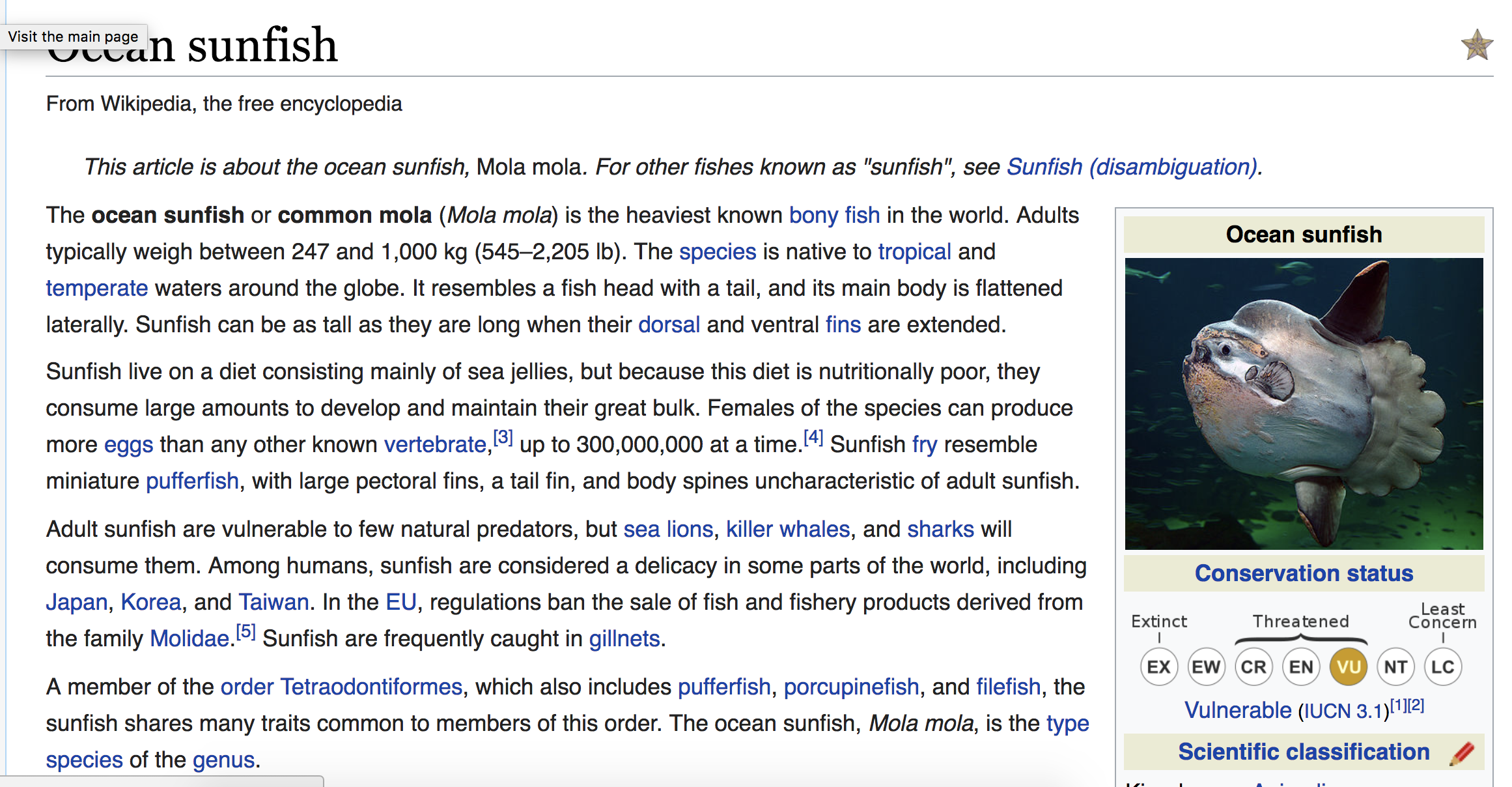A Wikipedia page detailing the ocean sunfish is prominently displayed. The page header includes an image of an ocean sunfish adorned with a gold star. The Wikipedia logo, a gray oval bearing the text "Wikipedia: The Free Encyclopedia," is present. The article commences with the name of the fish, "Mola Mola," highlighted in bold, followed by the phrase "for other fishes known as 'sunfish,' see sunfish (disambiguation)," also in blue and within quotation marks.

The primary focus of the text is on the ocean sunfish (Mola Mola), with the title "ocean sunfish" and "common mola" featured in bold. A notable claim follows: "It is the heaviest known bony fish in the world," with a hyperlink for further details. Typical adult weights, ranging from 247 to 1,000 kg (545 to 2,205 lb), are listed in parentheses. The species is indicated to be native to tropical and temperate waters worldwide, with both "tropical" and "temperate" linked in blue.

The right side of the page showcases an illustrative image of an ocean sunfish to complement the extensive information provided.